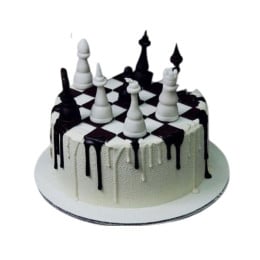The image depicts a meticulously detailed, digitally rendered chess-themed drip cake. Designed to resemble an actual chessboard, the cake features a top adorned with a black and white checkerboard pattern, complete with an array of chess pieces, some in black and some in white. The cake sits on a white cardboard platter and appears to be a single-layer creation, enhanced by alternating black and white frosting drips cascading down its sides, giving it a melting effect. This realistic and unique cake includes chess pieces such as a queen and a pawn prominently positioned on top, making it look as though one could begin a game of chess directly on the cake itself. The combination of the checkerboard design and the strategically placed chess pieces evokes a sense of both playfulness and elegance.